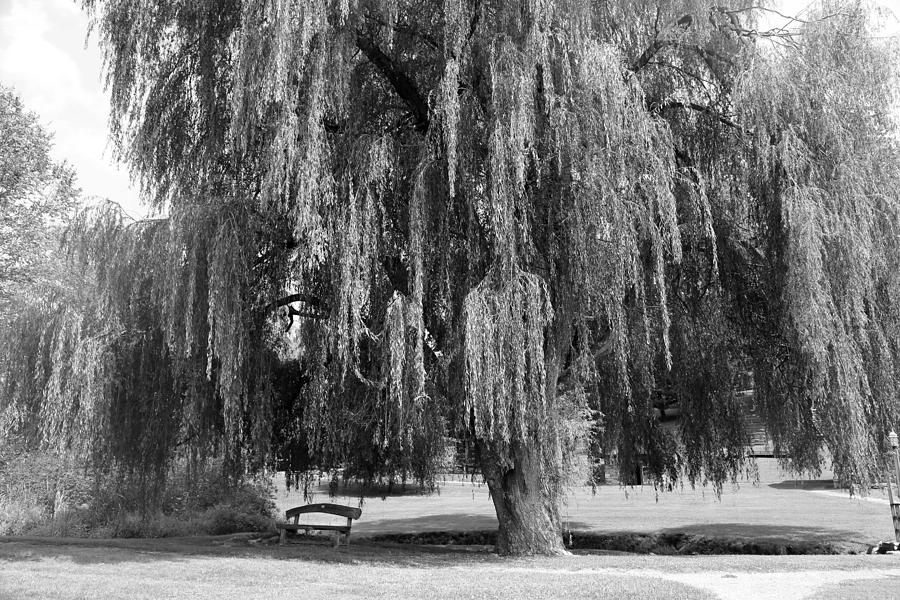This black-and-white photograph captures a serene park scene dominated by a majestic, ancient weeping willow tree at its center. The tree, with its thick base and cascading branches adorned with abundant, flowing foliage, occupies around 70% of the image. The weeping willow stands at the edge of a stream or small pond, creating a tranquil waterside atmosphere. Beneath its expansive canopy, to the left and the right, sits a small wooden bench with a carved back, inviting peaceful contemplation. Surrounding the tree, well-manicured green lawns stretch into the foreground and background, suggesting the meticulously kept grounds of a golf course. Smaller trees are also visible to the left of the main tree, adding depth to the composition. The photograph, devoid of any individuals or text, captures the timeless beauty and tranquility of the scene, with the grayscale tones emphasizing the contrasts and details of this professionally taken, realistic image.